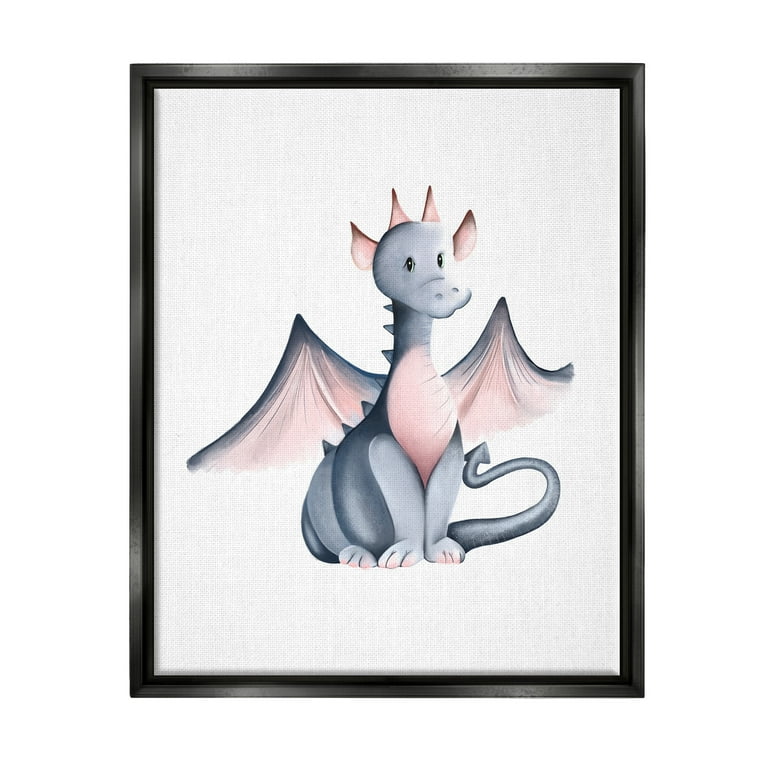This is a framed painting of a stylized dragon, depicted in predominantly gray and pink hues. The painting, potentially created with watercolors, pastels, or colored pencils, showcases the dragon against a solid white background. The dragon itself is primarily light gray or grayish-blue, with distinctive pink accents on its ears, horns, and the insides of its wings, which are outstretched and flared against its back. Its stomach and the fronts of its toes also share this pink hue. The dragon's body is further detailed with small, stegosaurus-like spikes running down its back, matching its gray body color. It has a tail curving out to the right, ending in a pointed, triangular tip. This creature faces slightly to the right, with black eyes and a rounded snout. The entire composition is elegantly enclosed in a thin, black picture frame, highlighting the clean and minimalist aesthetic of the piece.